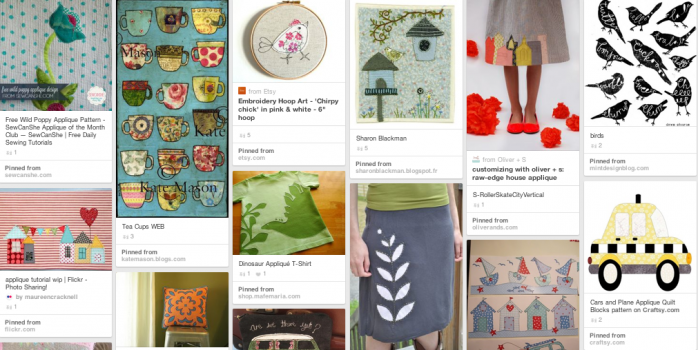The image showcases a collage of various embroidery works, displayed side-by-side possibly on a laptop screen. On the right-hand side, there is a woman wearing an embroidered skirt, with another woman beneath her also sporting detailed embroidery on her attire. The collage features embroidered t-shirts, pillows, and linens, demonstrating a range of intricate patterns.

One section highlights colorful designs on a tea towel adorned with various teacups. Another part of the image shows an antique quilt with the word "cars" and a police car embroidery. Additional embroidery pieces include scenes with boats on the water and beach huts, as well as vibrant birds with diverse designs perched on bird houses.

A prominent detail is an embroidery hoop with a beautifully crafted bird, emphasizing the theme of textile embellishments. The overall collage vividly exhibits the artistry and versatility of embroidery on different materials and objects.